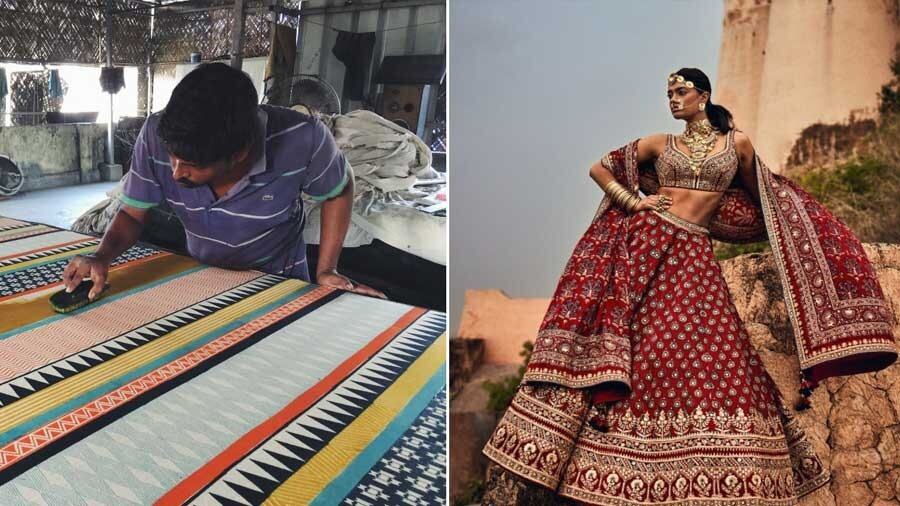The image is a side-by-side composition of two photographs illustrating a thematic contrast between creation and final product. The left photograph depicts an Indian man in a blue and white striped shirt, engrossed in his work at a rough-hewn workshop. He bends over a table or counter laden with various brightly colored fabrics, featuring geometric patterns in orange, black, white, blue, and yellow. The man is holding a hand brush over one piece of fabric, seemingly treating it, with a smartphone also placed on the table. The workshop background reveals a rustic setup with a metal wall and a thatched upper section, alongside a pile of additional fabric. 

The right-hand photograph captures an elaborately adorned Indian woman posing against a backdrop of red rock formations. She is impeccably dressed in traditional attire, wearing a red bikini-style top with intricate red and gold patterns, along with a long red skirt decorated with intricate gold and gray designs, and a gold-bordered hem with arched motifs. Her ensemble is complemented by a large red, white, and gray shawl. The woman is richly accessorized with head jewelry, a nose ring, earrings, a gold neckpiece, numerous gold-colored bracelets, and rings. She stands confidently with her right hand on her hip, striking a pose that showcases the detailed craftsmanship of her attire. Behind her, the scene includes tall stone structures in light brown hues, adding to the dramatic effect of the photograph. Together, the photos juxtapose the meticulous process of fabric treatment with the resplendent final product showcased by the elegantly dressed model.